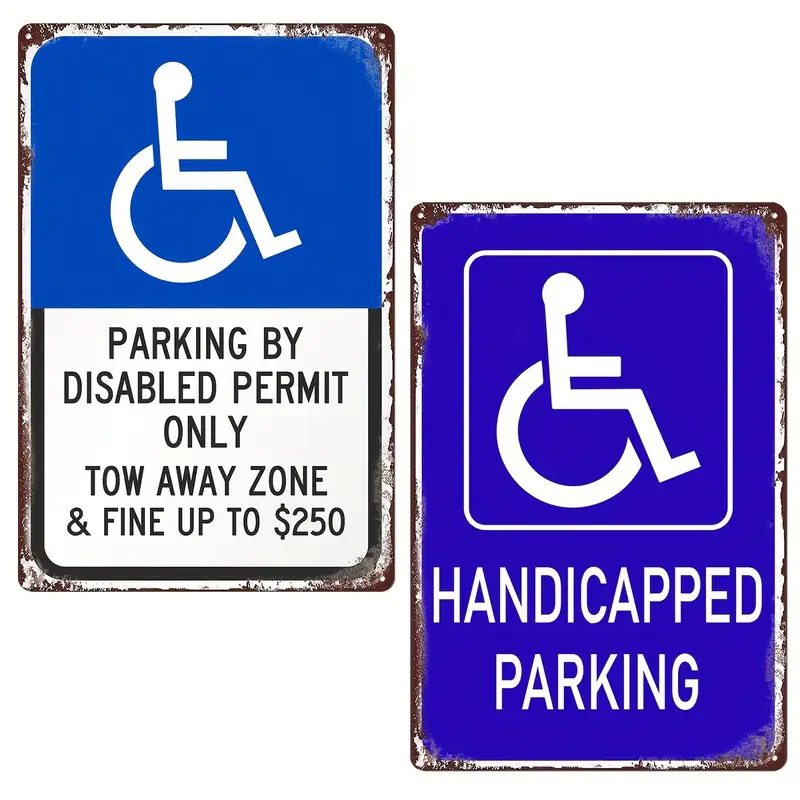The image displays two vertically rectangular, metal handicap parking signs, arranged side by side, with a noticeable silver border that is rusted and worn. The signs appear weathered, with paint chipping away at the edges. 

The sign on the left is divided into two sections: the upper half features a blue background with a white stick figure of a person in a wheelchair, while the lower half has a white field with black text that reads, "Parking by disabled permit only, tow-away zone, and fine up to $250." 

The sign on the right presents a simpler design, with an entirely blue background showcasing the same white stick figure of a person in a wheelchair, accompanied by the text "Handicapped Parking" below the symbol.